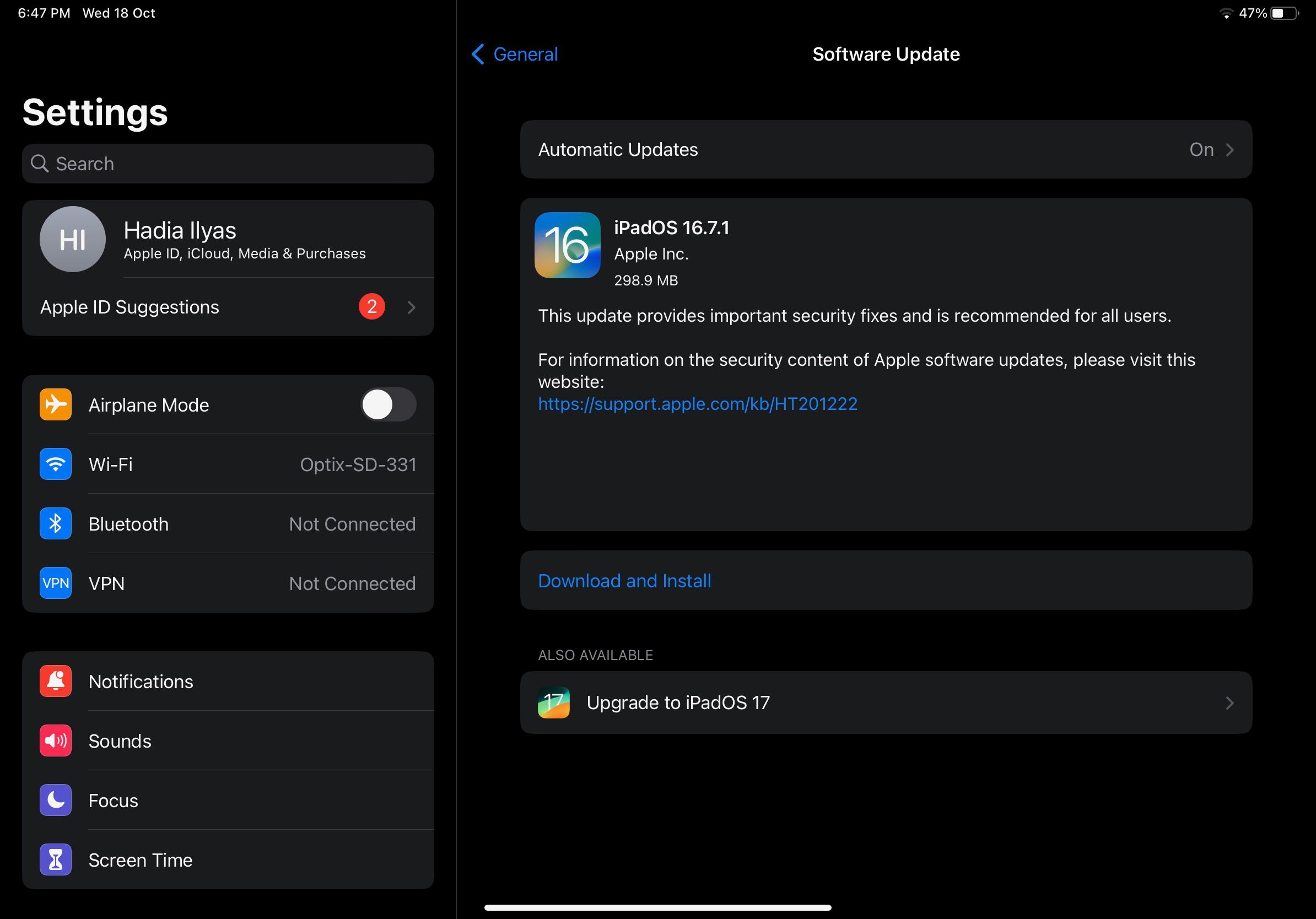**Descriptive Caption:**

The image displays a screenshot of an iPad settings page, captured at 8:47 PM as indicated at the top. The background of the interface is black. At the very top, a search bar is visible beneath the title "Settings." Below this, a gray circular icon labeled "HI Hattie alias Apple iCloud, Media, and Purchases" is shown, along with a notification in red text stating "Apple ID Suggestions: 2."

To the right is a right-pointing arrow, indicating further options. The page shows various sections with details:

- **Airplane Mode**: Indicated by a yellow airplane icon, is turned off.
- **Wi-Fi**: Connected to a network named "OPTIX-SD-331."
- **Bluetooth**: Not connected.
- **VPN**: Not connected.
- **Sections**: Notifications, Sounds, Focus, and Screen Time.

Further down the page, a section titled **Software Update** is shown, with a left-pointing arrow labeled "General." It mentions that automatic updates are on, and the current version is **iPadOS 16.7.1**. The update, sized at 293.9 megabytes, is from Apple Inc. and provides important security fixes, recommended for all users. A square with the number "16" is also shown beside this information.

A note directs users to visit a website for more information about the security content of Apple software updates: [Apple Support HT201222](https://support.apple.com/en-us/HT201222). The options "Download and Install" and "Upgrade to iPadOS 17" are displayed at the bottom of the page.